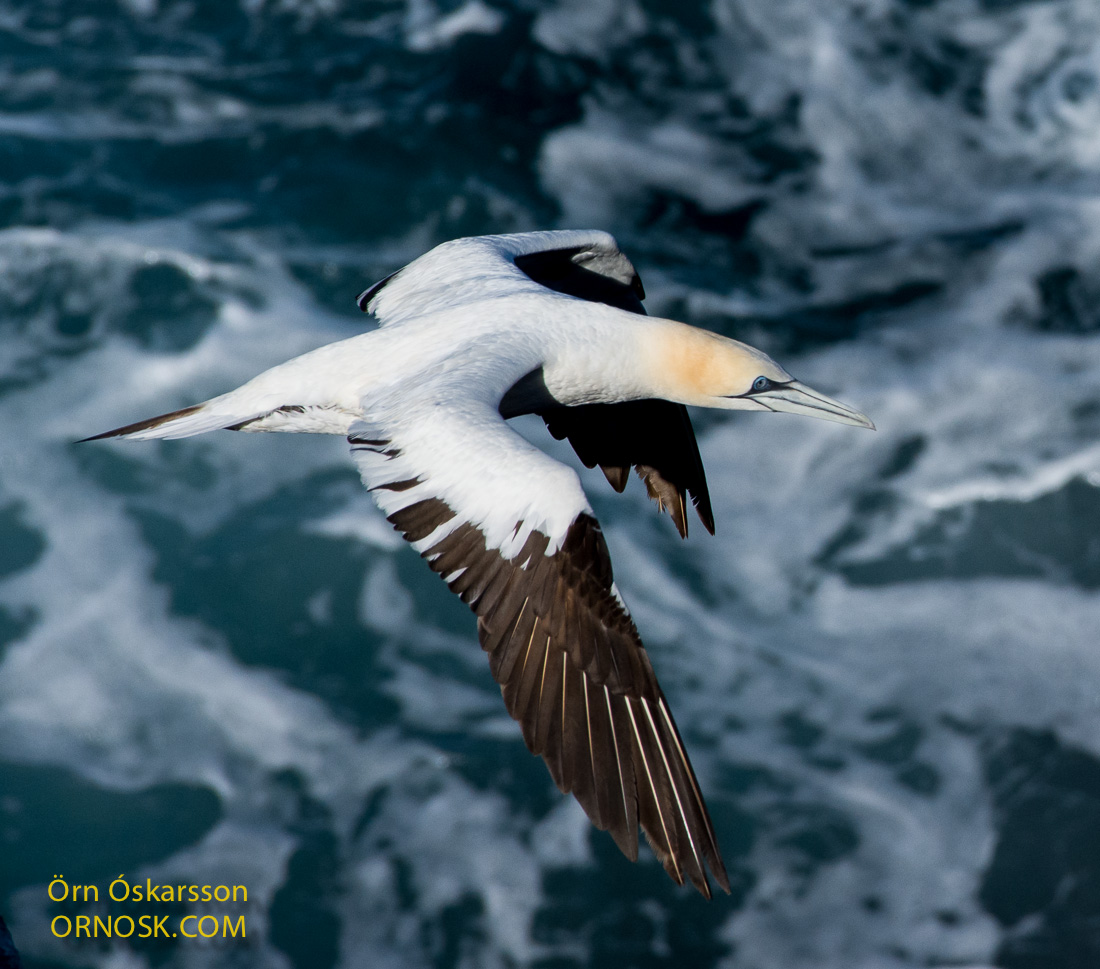The image features a large bird in mid-flight, captured from an aerial perspective, soaring above a chaotic, dark gray expanse of water dotted with wavy whitecaps and sea foam. The bird's plumage is primarily white, with its head and body predominantly white, accentuated by dark brown wing tips and edges. Notably, the bird has an orangey hue around its cheeks and black markings around its blue eyes. Its distinct features include a long white bill and a pointed tail with a combination of black and white feathers. The bird's expansive wings are captured with the tips down, creating a dynamic sense of movement. On the lower left-hand corner of the image, the text "ORN OSKARSSON" is written in yellow, followed by the website "ORNOSK.com."